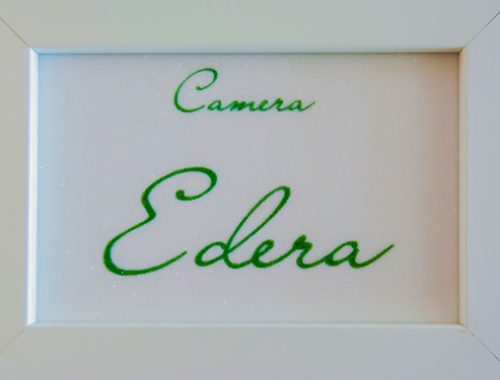This photograph captures a white, square picture frame displaying a handwritten message. The frame, made of wood, reveals thin borders on the left and right sides and thicker edges on the top and bottom. The background within the frame is white or cream, creating a clean canvas for the elegant, green cursive text. The text reads "camera Edera," with "camera" written smaller and above "Edera." The image appears incomplete due to being cut off on the left and right, and there is noticeable shadowing on the right, suggesting a light source from the left. No other objects or elements are present, and the overall quality is medium despite the cropping.